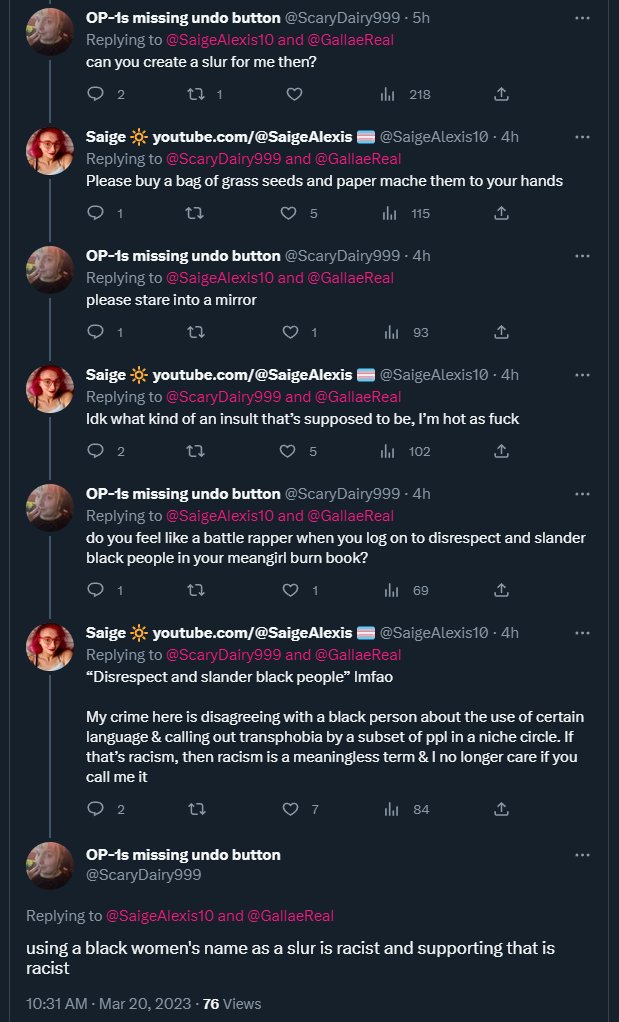A screenshot depicts a chat from an unidentified app with a black background, featuring a conversation between two users. The first user's profile photo, displayed on the left, is of an individual with bangs whose gender cannot be determined. This user, "miss an undo button" (username "op_ones"), has posted a message five hours prior, replying to "sagealexis10" and "gallerioreal," asking, "Can you create a slur for me then?"

The second user, "sageyoutube.com" (username "sagealexis"), likely a woman with red hair, responded with, "Please buy a bag of brass seeds and papier-mâché them to your hands."

The conversation shows a back-and-forth exchange between "op_ones" and "sagealexis," culminating in "op_ones" stating, "Using a black woman's name as a slur is racist and supporting that is racist." This final message includes a timestamp of 10:31 AM on March 20th, 2023, and has accrued 76 views.